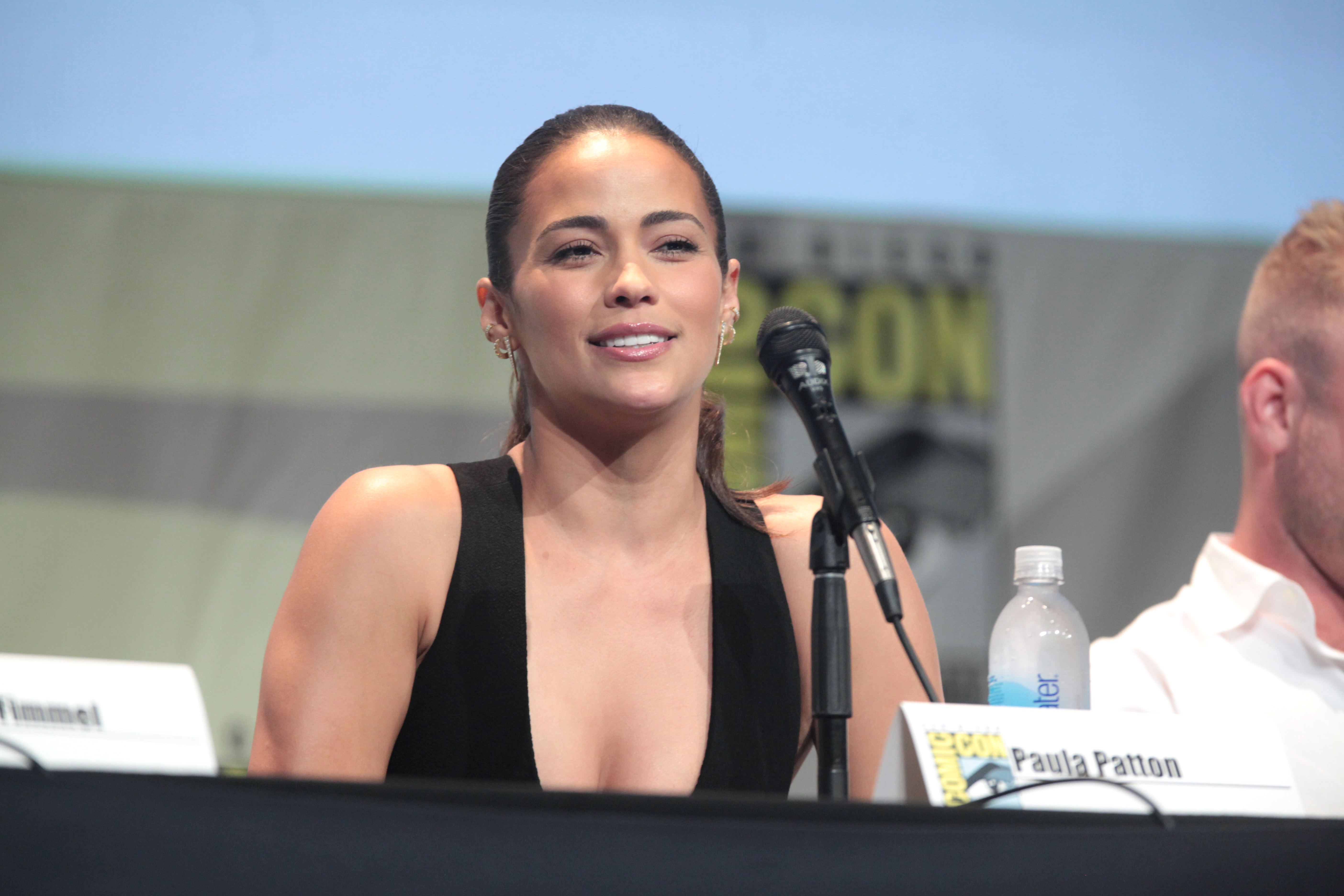This image features the actress Paula Patton at a San Diego Comic-Con event. Paula is seated behind a podium adorned with a white name plaque displaying her name in black letters. She is wearing a black, sleeveless top that is fairly low-cut, showing some cleavage. Her hair is pulled back into a ponytail, and she is accessorized with golden dangly earrings, red lipstick, and a noticeable amount of makeup. In front of her is a black microphone on a stand and a clear, unopened water bottle, which might be Smartwater, placed next to the name card. Paula is smiling, possibly engaged in answering a question or preparing to respond. To her left, another name card is partially visible, and to her right, a man in a white polo shirt can be seen. The recognizable San Diego Comic-Con logo is visible in the background.